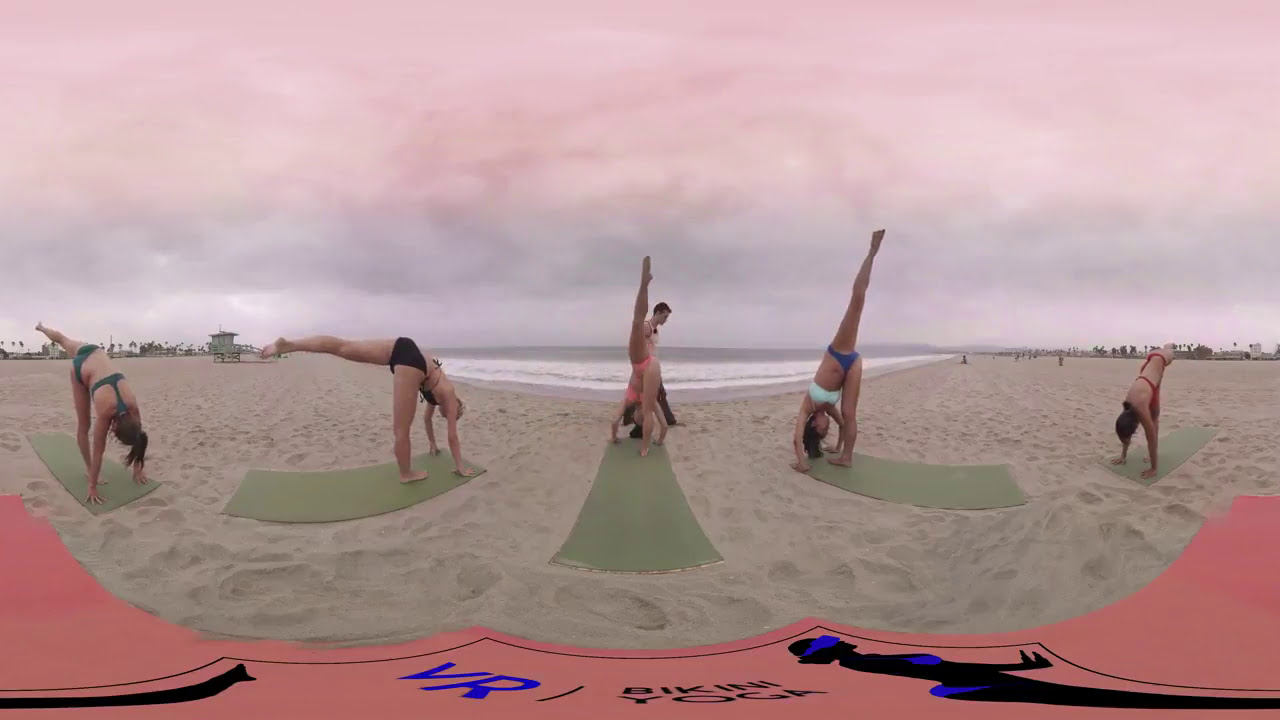In this detailed image, five women are engaged in various yoga poses on a sandy beach under an overcast, gray sky. They are all dressed in bikini swimsuits and positioned on sage green yoga mats. From left to right, the first woman is in a green bikini, the second in a black one, the third in pink, the fourth in a green top with a blue bottom, and the fifth in red. Each woman displays an inverted pose with their palms planted shoulder-width apart on the mat, their torsos bent forward, and one leg lifted in the air at hip height or higher. Behind them, we can see the ocean stretching towards the horizon, with gray and pink clouds filling the sky. The overall scene gives a slightly distorted, rounded appearance, likely due to the use of an ultra-wide or 360-degree lens, which also makes a pink banner at the bottom appear scalloped. A man’s head is visible in the background, walking along the beach behind the woman in the pink bikini.